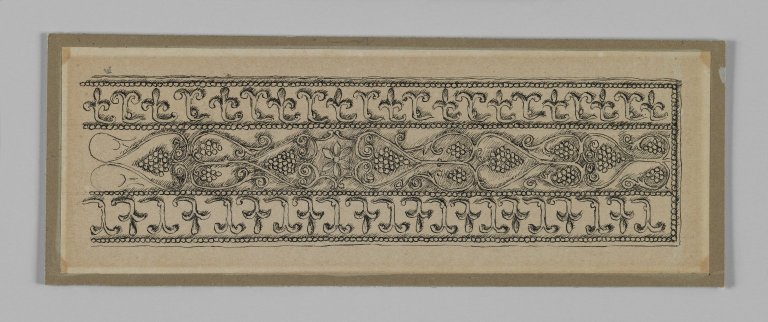The image depicts a horizontal, landscape-style wall hanging with a thin brown border set against a gray-blue wall. The artwork inside features a light tannish background. Across the top and bottom, there are repeating symbols resembling non-capitalized T's and Y's, interspersed with a border made of circular stitching. The centerpiece of the hanging is an intricate design that appears to represent a grapevine with clusters of grapes, extending horizontally. This central motif is outlined by heart-shaped patterns. Additional rows of circular stitching border these elements above, below, and on the right side, but not on the left. The entire piece resembles a detailed label, possibly created with fine brushes or pencil, emphasizing detailed artistry and elaborate dot patterns throughout.